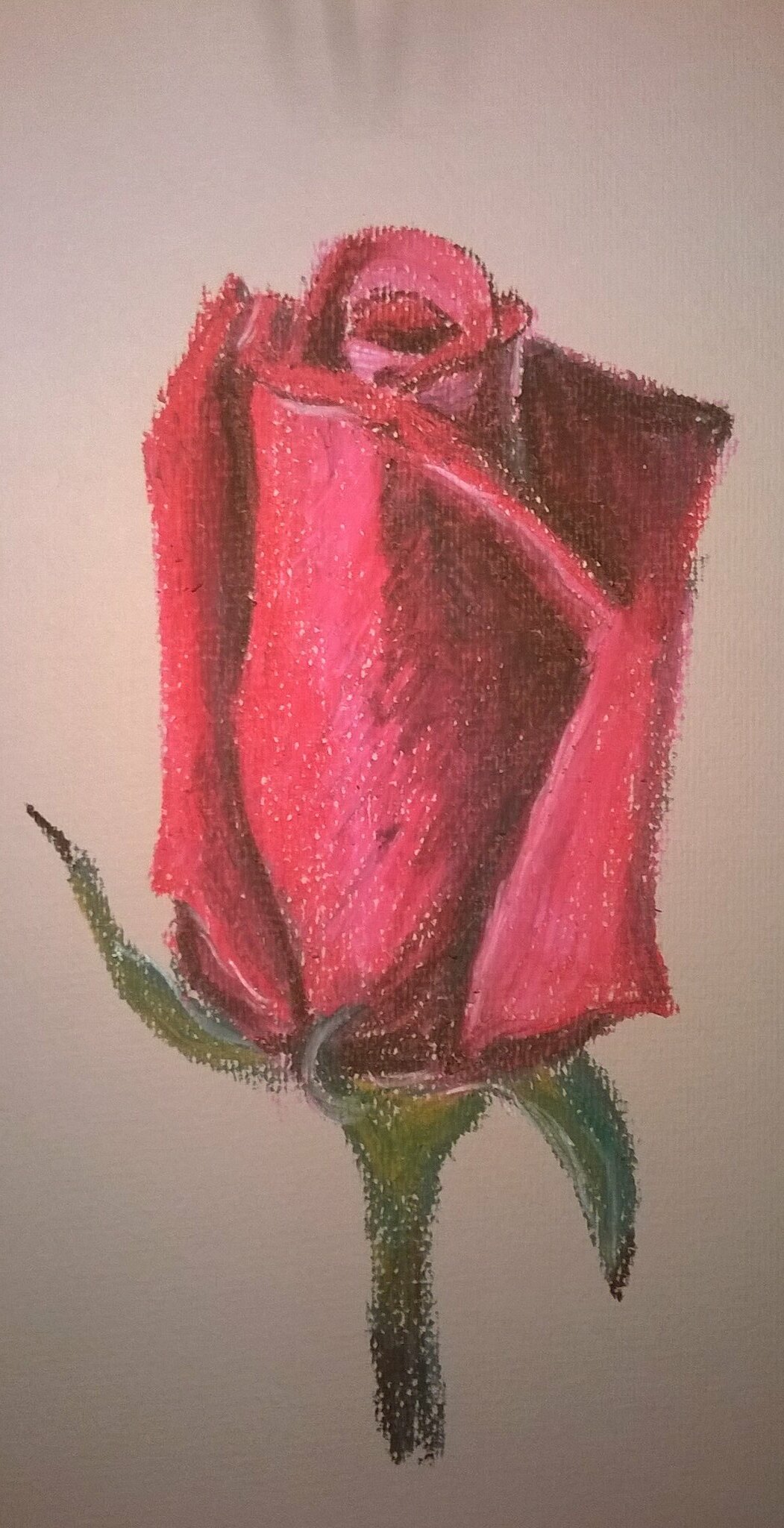The image showcases an artistic depiction of a rose that appears to be created using pastels, characterized by its fine lines and shadings. The rose, which is in the early stages of bloom, has outer petals that are starting to open while the inner petals remain tightly held together. The flower displays a rich palette of dark red, light red, and a touch of pink at the top, adding a delicate touch to the illustration. The upright rose features a dark green stem with pointed leaves; one points upwards and another downwards, indicating a natural, slightly curved posture. The composition is set against a light brown or off-white background, creating a subtle contrast that highlights the rose's vibrant colors. Additionally, the upper part of the background includes a shadow-like effect, contributing depth and a darker tone to the overall image.